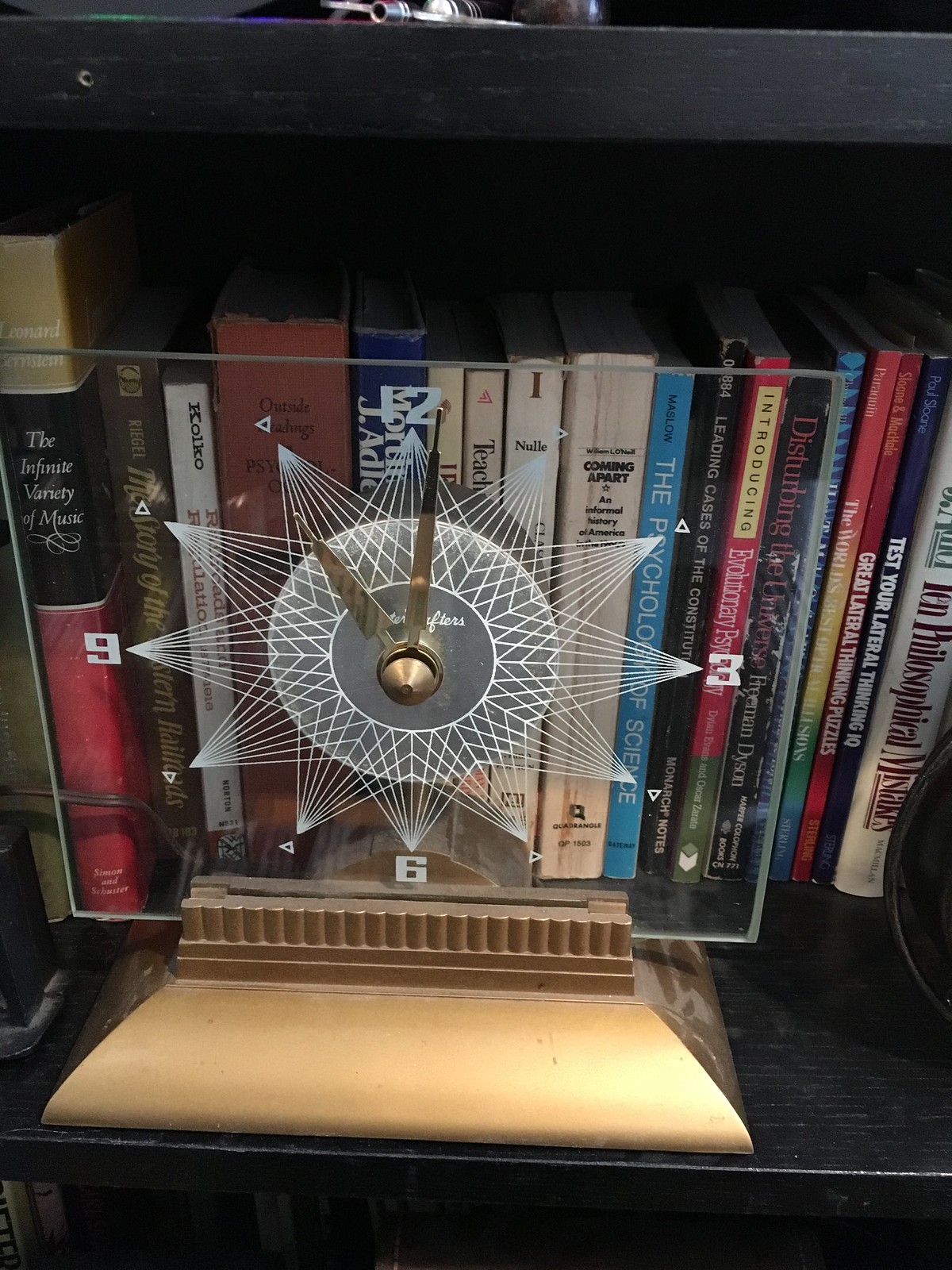This color photograph depicts a section of a black-painted wooden bookshelf lined with a diverse collection of at least 10 to 15 books of varying thicknesses. Among the books, some have red and black spines with gold lettering, while others display white spines with red text. Distinct titles visible include "The Infinite Variety of Music," "Coming Apart," "Psychology of Science," and "It's Your Lateral Thinking."

In front of the books, an intriguing clock, designed to resemble a compass, stands out. The clock face is etched in clear glass, with a complex star pattern formed by numerous fine lines. The numbers 12, 3, 6, and 9 are marked at the cardinal points; other positions are indicated by small triangles. The clock boasts gold hands, which point to just after 11 o'clock—though another description mentions a different time. The clock rests on a light brown or matte gold base, providing a stylish contrast to the books behind it.